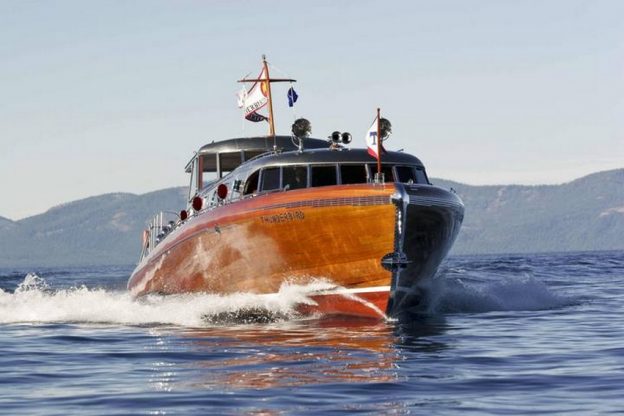This image captures a striking depiction of a medium-sized motorboat advancing toward the camera, angled slightly to the right, through a water body that could be either a sea, lake, or cove. The boat’s hull is constructed from richly-grained, polished brown wood, exhibiting various shades and darker grain details. The upper structure of the boat, which includes a cockpit or cabin area, is composed of bright silver metal, giving it a retro appearance reminiscent of 1970s or 80s designs. It features two distinct decks: the lower one is mostly enclosed but allows walking around the edge in the open air, while the upper section is more open and characterized by numerous windows. Flying from two flagpoles, which match the wooden color of the deck, are multiple flags billowing in the wind. Additionally, the boat is fitted with railings at the back. A pronounced bow wave is seen on the left side of the photograph (right side of the vessel), showing its speed and dynamic movement through the water. In the background, there is an island or landmass with very tall terrain, including mountains or significant hills, under a clear sky, completing the detailed maritime scene.